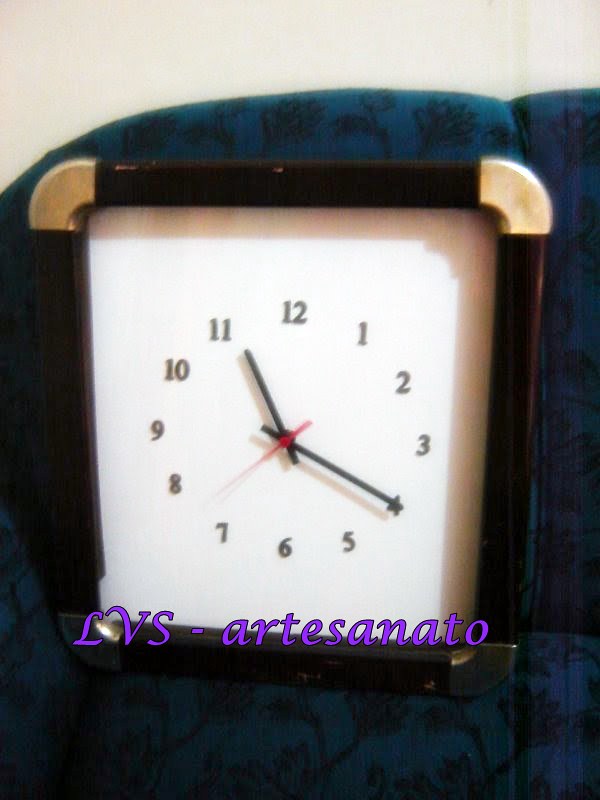A detailed photograph captures a square clock resting on a blue couch adorned with black floral and shrubbery designs. The clock features a black border with brass or steel corner accents, giving it a sleek, modern look. Its face displays large, clear numbers without any intermediate dashes and includes hour, minute, and second hands. The time shown is 11:20, with the second hand positioned just past the 35-second mark. In striking purple lettering over the clock face, the text "LVS-Artenz-Santanato" is prominently displayed, adding an intriguing layer to the visual composition.